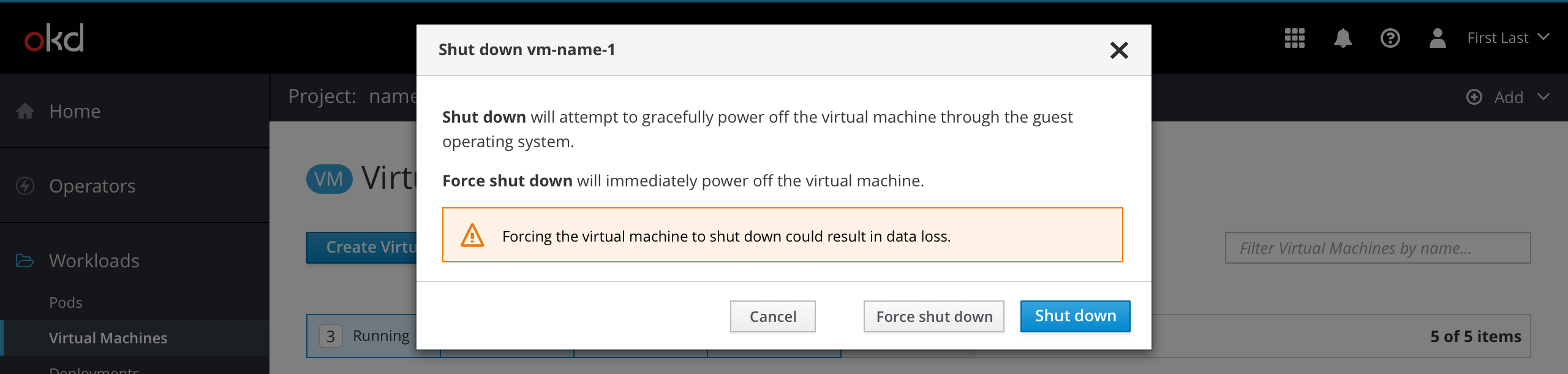In the center of the page is a prominent pop-up titled "SHUTDOWN VM NAME 1" in black text on a white background. The main message indicates two options: "SHUTDOWN" will gracefully power off the virtual machine via the guest operating system, while "Force SHUTDOWN" will immediately cut the power, potentially causing data loss. This warning is emphasized with a brown and orange outline and an orange warning triangle with an exclamation mark.

At the bottom right of the pop-up are three buttons: "CANCEL" and "FORCE SHUTDOWN" in grey, and "SHUTDOWN" in blue.

In the background, the left side of the page features a black section with the label "OKD", where 'O' is red and 'K' and 'D' are grey. Below this are navigation options including "HOME," "OPERATORS," "WORKLOAD," "PORT," and "VIRTUAL MACHINES," alongside a project name and a blue button labeled "VM VIRTUAL MACHINES."

To the left of the pop-up, there is the option to "CREATE VIRTUAL MACHINE." Below this are status indicators showing three running instances. On the right side, a search box reads "FILTER VIRTUAL MACHINE BY NAME."

Above all this, a grey toolbar houses several icons: "CREATE VIEW," "NOTIFICATION," "HELP," and "PROFILE ICON," followed by a "HEAD" button, all in grey.